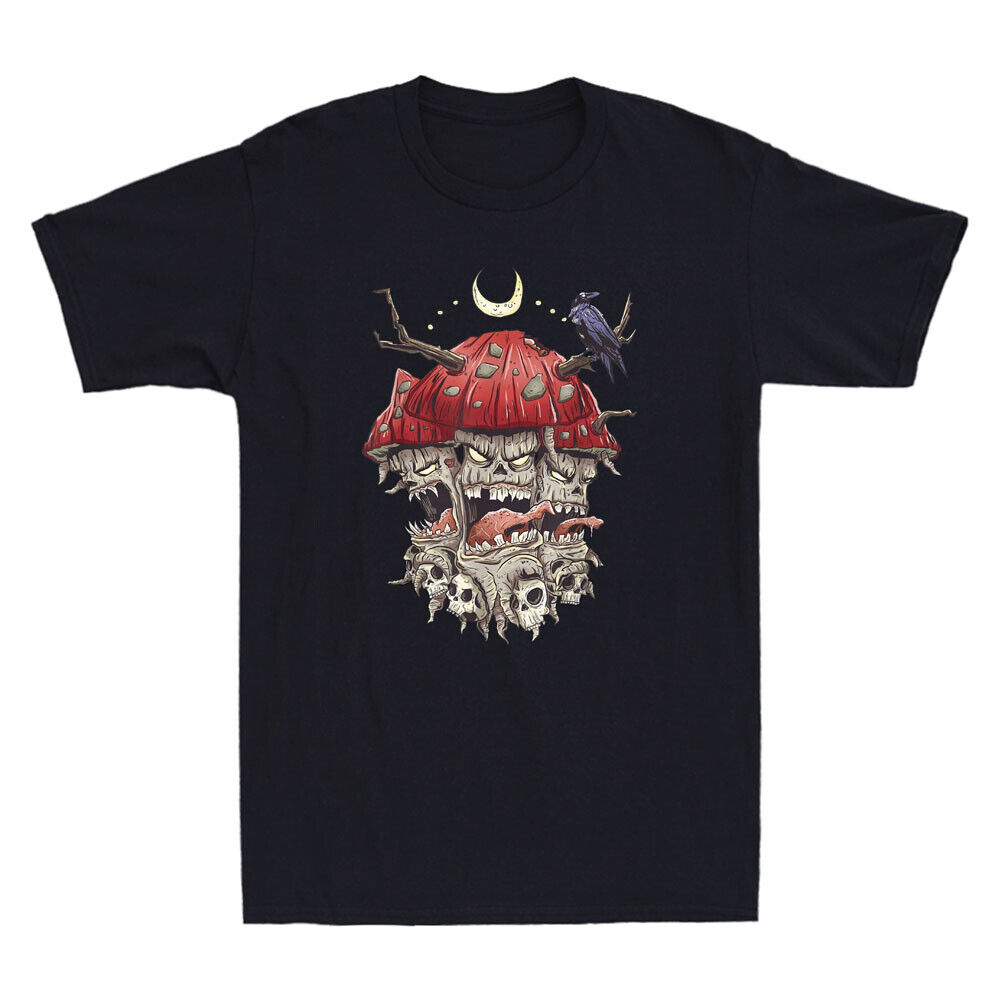This image showcases a black T-shirt laid out flat against a white background, emphasizing the detailed illustration on its front. Dominating the design is a mushroom scene: at the top, a small yellow crescent moon faces upward. Below it, a prominent red-capped mushroom is central, with branches extending from each side. A purplish bird perches on the right branch. The mushroom's stem features a haunting face with yellow eyes, an open mouth displaying white teeth, and a yellow tongue. Flanking the central mushroom are two identical red-capped mushrooms, each with a similarly eerie face in their stems. At the bottom of the design, white skeletons are visible. The T-shirt's striking imagery stands out vividly against its solid black background.